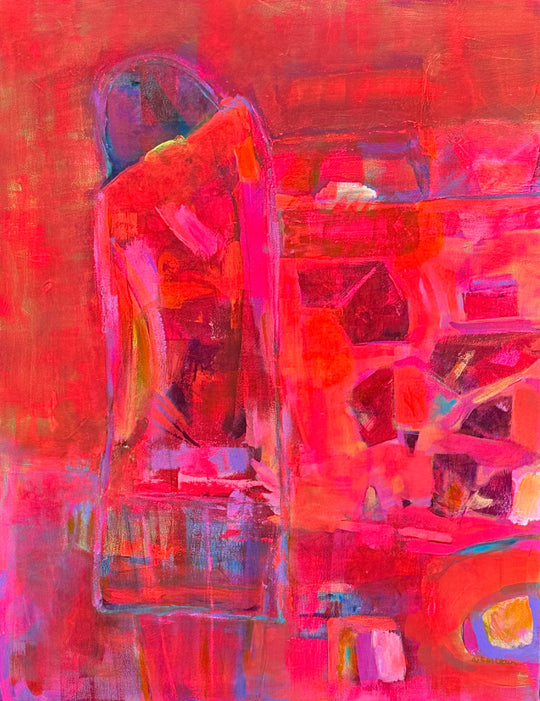This image is a modern, oil painting rendered in portrait mode with a detailed interplay of shapes and colors. Dominated by shades of red, pink, dark blue, and purple, the painting employs light blue outlines to define its features. At the center, there appears to be a figure, likely a woman, discernible from the dark hair and what resembles a dress or skirt. Some interpret the figure as possibly wearing a hat. 

She stands in front of what seems like a dressing room mirror or a bar table, as there are various items taped to or placed around the mirror and table, suggesting personal or work-related surroundings. The background comprises a collage of shapes—squares and triangles—that are open to interpretation, possibly representing books, shelves, or miscellaneous clutter. The style is predominantly abstract, blending a mixture of bright and dark tones to create a vibrant yet somewhat ambiguous scene. The artist's name is inscribed in the lower right corner, though it is not legible.